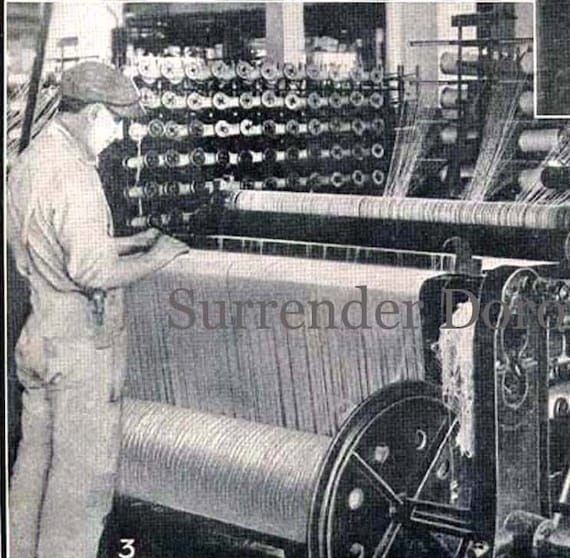The image is a black and white, vintage-style depiction, possibly a textured photograph overlaid with crosshatched pencil lines, of an industrial scene from the early 1900s. It features a three-quarter view of an old weaving machine, likely used during the turn of the century. On the left side of the image stands a man dressed in overalls, a long-sleeved shirt with the sleeves rolled up, and a newsboy style cap. He is intently looking down and working with the large industrial loom, where threads from multiple feeder spools in the upper right corner converge into the machine. Finished fabric is collected on a spool at the bottom of the loom. Behind him, there's a wall filled with large reels or spools of yarn or thread, indicating a busy, bustling factory environment. The scene is primarily rendered in shades of gray and white, emphasizing its vintage nature. Superimposed over the middle of the image, there are words in a modern font that read "Surrender Dorothy," though the latter part of the text trails off the right edge of the image.